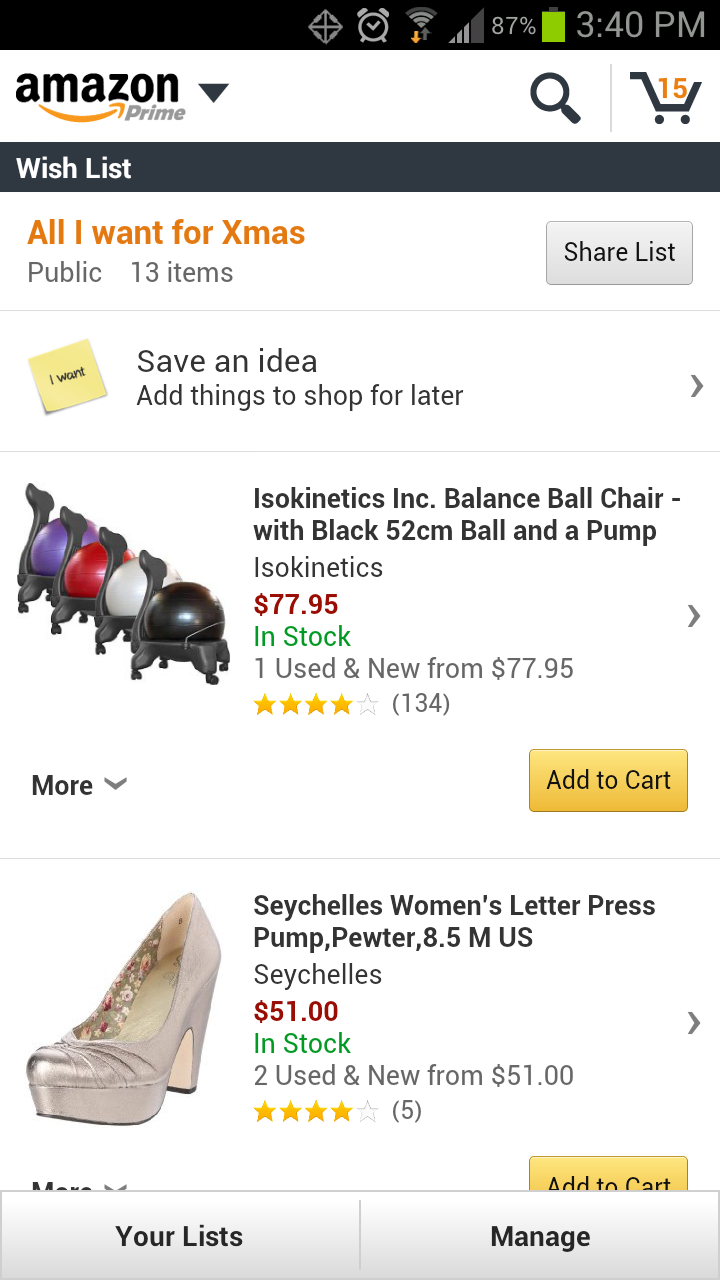This detailed image shows an Amazon website interface formatted for a mobile phone.

### Top Section:
- **Black Bar:**
  - Center-right: Mobile icons including a clock, Wi-Fi signal, cellular signal strength, 87% battery life, and a "3.4 TPM" indicator.

- **Amazon Header:**
  - Amazon logo and Amazon Prime label.
  - Search box.
  - Shopping cart with 15 items indicated.

### Middle Section:
- **Black Banner:**
  - Left: "Wish List" in white text.
  - Center: "All I Want for Xmas" in orange, labeled as public with 13 items.
  - Right: Grey button to "Share List."

- **Wishlist Explanation:**
  - "Save an Idea" feature allows users to add items for later shopping.
  - A small yellow post-it note on the left side reads "I Want."

### Item Listings:
1. **First Item:**
   - **Product:** Isokinetics Inc. Balance Ball Chair with black 52cm ball and pump.
   - **Brand:** Isokinetics.
   - **Price:** £77.95.
   - **Availability:** In stock.
   - **Additional Details:** One used and new option available for £77.95. Four-star rating from 134 reviews.
   - **Visuals:** Images of the chair in purple, red, white, and black.
   - **Actions:** Yellow "Add to Cart" button on the right side.

2. **Second Item:**
   - **Product:** Seychelles Women's Leather Press Pump.
   - **Color and Size:** Pewter, 8.5 US.
   - **Brand:** Seychelles.
   - **Price:** $51.
   - **Availability:** In stock.
   - **Additional Details:** Two used and new options available for $51. Four-star rating from five reviews.
   - **Description:** Metallic beige high-heeled court shoe with a platform front and cut-out design. The heel is high but not extremely pointy like stilettos.
   - **Actions:** Partially obscured yellow "Add to Cart" button on the right side.

### Bottom Section:
- **Navigation Tabs:**
  - Left: "Your Lists" within a light grey rectangle.
  - Right: "Manage" within the same color rectangle.

This cleaned-up and descriptive caption provides a comprehensive overview of the image, detailing every observed element on the Amazon mobile interface.